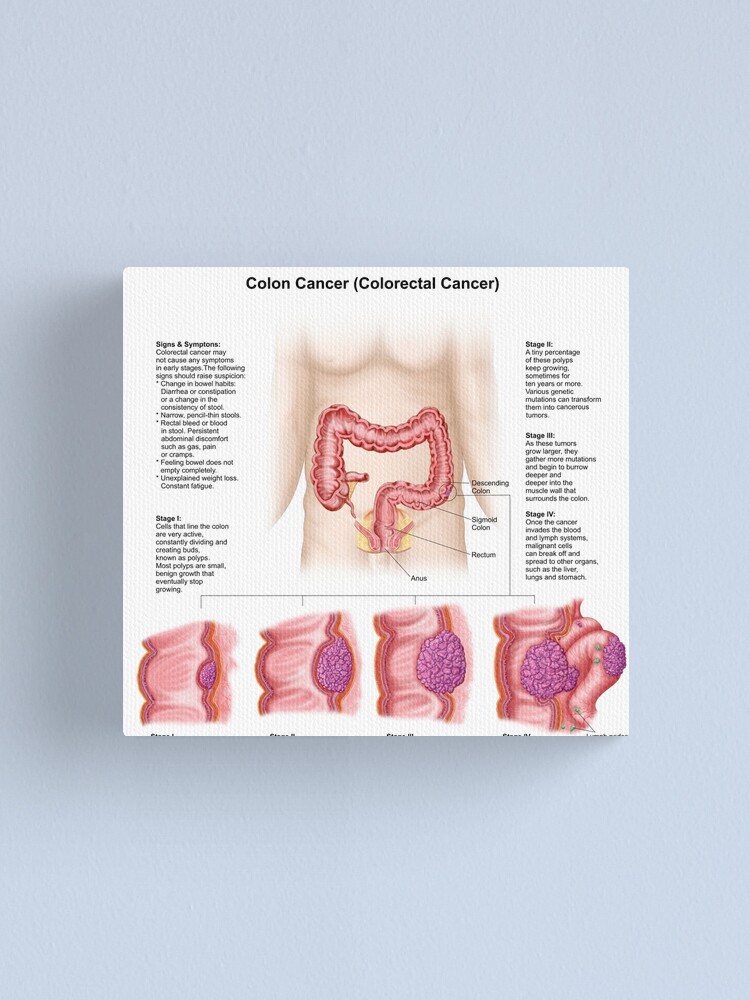The image depicts a rectangular poster on the topic of colorectal cancer. It is set against a monotone, slate-gray background and shows a white, canvas-like square in the center. The dimensions of the gray background are approximately five to six inches high and four inches wide, whereas the white square is about two inches high by two inches wide with slightly rounded corners.

At the very top of the white square, bold black text reads "Colon Cancer (Colorectal Cancer)." Below this title, a detailed medical illustration of a male torso showcases the large intestine, depicted in shades of pink and red. The image includes identifiers for various parts of the colon: descending colon, sigmoid colon, rectum, and anus. Black lines extend from these parts to very small labels, which are not legible.

To the left side of the torso image, the section is labeled "Signs and Symptoms," and underneath it says "Stage 1." On the right side, there are more labeled sections: "Stage 2," "Stage 3," and "Stage 4," each followed by small, unreadable text. These sections describe the progression stages of colorectal cancer.

Toward the bottom of the white square, there are four smaller diagrams depicting close-up views of the colon. Each diagram illustrates the sequential growth of a tumor within the colon lining. The tumors, colored in purple, increase in size with each subsequent image, contrasted against the light pink background of the intestine.

Overall, the poster provides a comprehensive overview of colorectal cancer, detailing the stages of tumor development while being heavily annotated, although much of the finer text remains unreadable from the image.